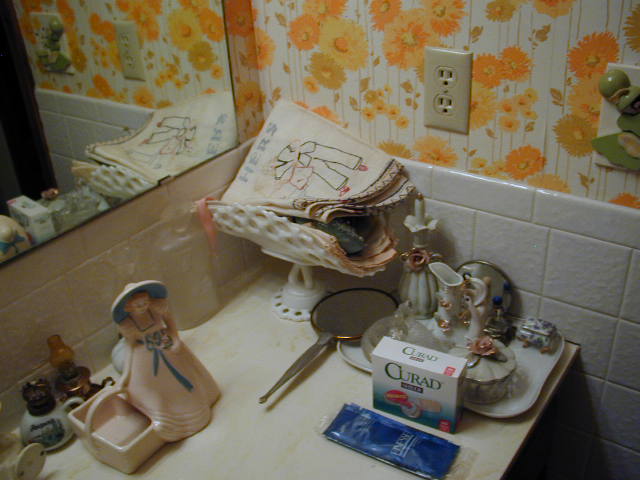This photograph captures a quaint bathroom setting featuring a beige or off-white countertop adorned with an array of intriguing items. On the right side of the countertop, there's a small collection of perfume bottles; one of them is white with a brown cap, while the other is a brown bottle with an amber-colored cap. A delicate ceramic sculpture of a woman wearing a pink dress with a blue bow and a matching blue and pink hat, holding a pink basket, adds a touch of whimsy to the scene.

Resting beside the perfume bottles is a handheld mirror with a silver frame and a gold border around its round mirror at the top. A box of "Curate" band-aids lies nearby, alongside a mysterious blue rectangular package. Additionally, a ceramic tray holds a variety of other ceramic trinkets in off-white hues, some adorned with pink flowers, in various rectangular and circular shapes.

The wall on the right side of the photograph features white tiles, while the left side appears slightly off-white, possibly due to shadowing. The upper right corner reveals a glimpse of white wallpaper embellished with bright orange and green sunflowers. A mirror on the left-hand wall reflects many of these items, offering a mirrored view of the charming arrangement on the countertop.